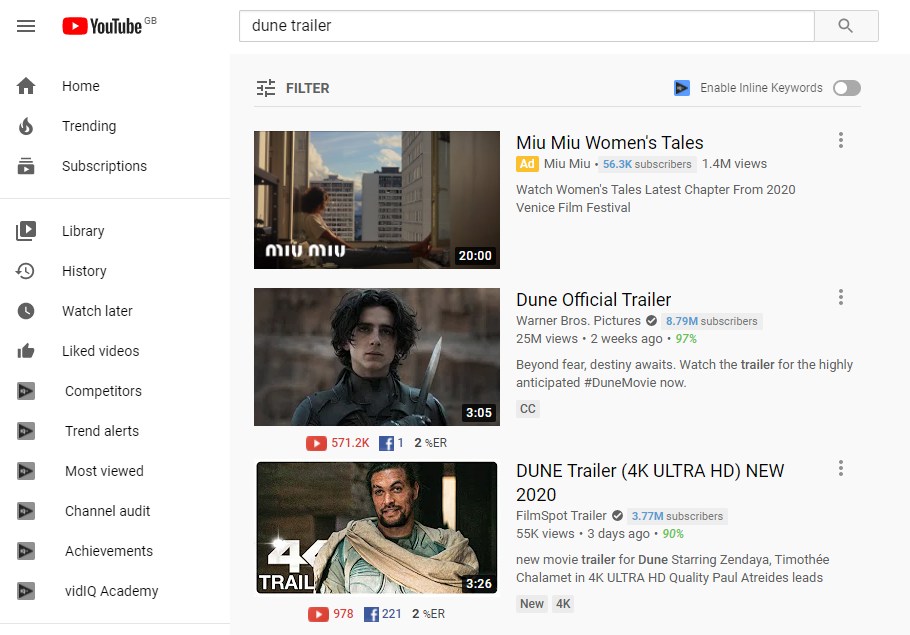The image displays a YouTube search result page for the query "Doom trailer." The first result is clearly marked as an advertisement. The second result is the official trailer for the "Doom" movie, uploaded by Warner Brothers, featuring a description that reads: "Beyond Fear, Destiny Awaits. Watch the trailer for the highly anticipated #Doom movie now." The third result, which appears to have been posted more recently (three days ago), is a 4K Ultra HD video. This specific video includes additional details indicating it may be from a different country, as evidenced by the "GB" notation next to the YouTube logo, suggesting geographically tailored search results. Each video listing includes the number of subscribers of the uploader and a verification badge. Additionally, the description for the third video highlights the full 4K Ultra HD quality and mentions key actors Zendaya and Timothee Chalamet, noting that "Paul Atreides leads." On the left-hand side of the screen, the traditional YouTube navigation bar is visible, featuring various buttons for navigating different sections of the platform.